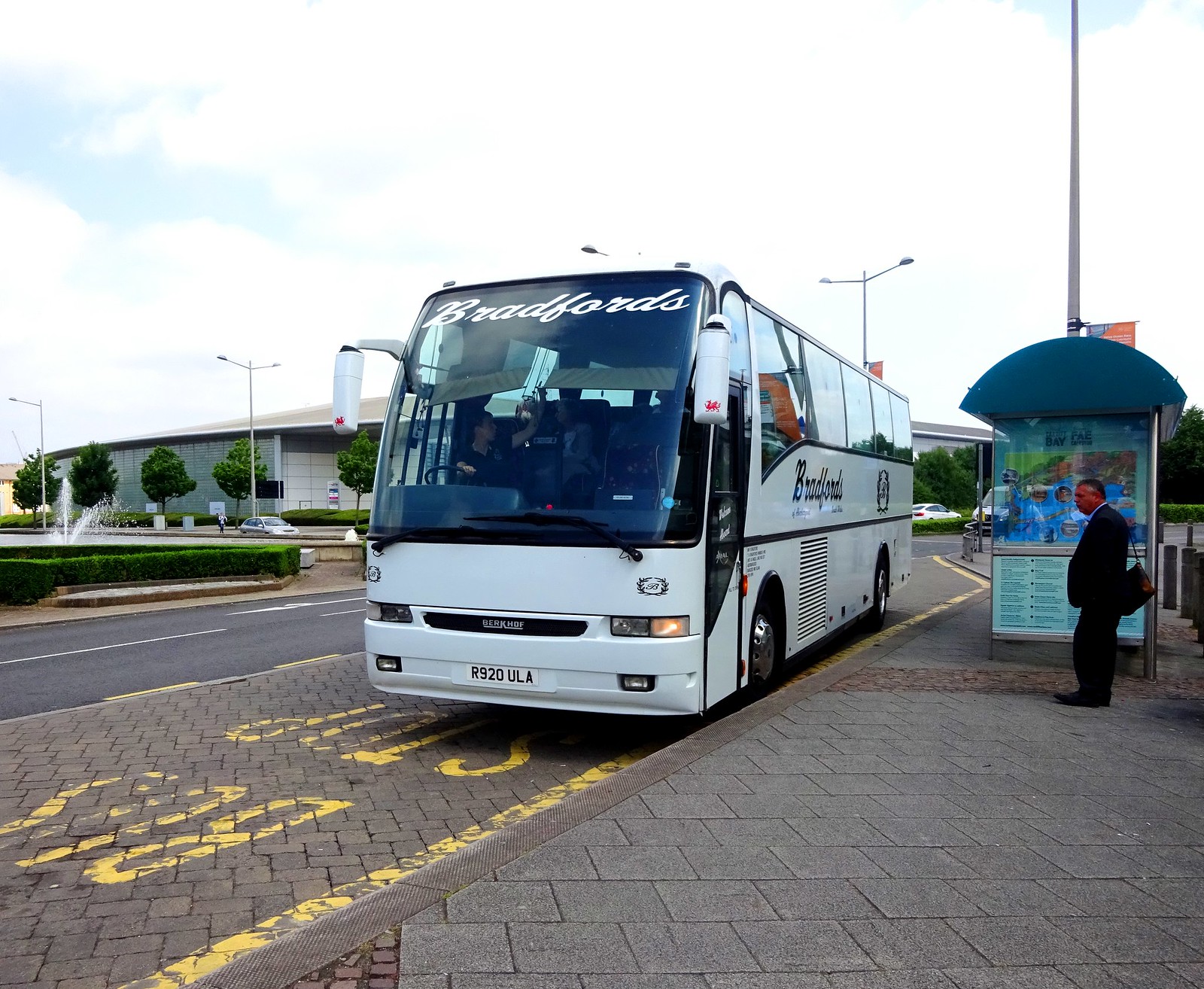The photograph captures an outdoor scene at a bus stop in daylight with a significant amount of white clouds in the sky. The clean white bus, labeled "Bradford's" across both the top of its windshield and on its side, is parked by the curb alongside the bus stop. The bus is turned on, with its lights illuminated. A middle-aged man dressed in a black suit stands on the extreme right of the image, facing left. He holds a brown shoulder bag and waits under a metal canopy with a dark green arc-shaped roof, supported by metal structures.

The bus has large windows, especially at the front, and there are two people visible inside: the driver in a black t-shirt and a passenger in a gray jacket or sweatshirt. Yellow letters spelling "BUS STOP" mark the pavement in front of the bus. The surroundings feature a mix of urban and natural elements, including a gray sidewalk, hedges, a fountain, and a row of green trees leading up to a round, possibly stadium-like building in the distance. Street lights are scattered throughout the area, completing the bustling yet serene cityscape.